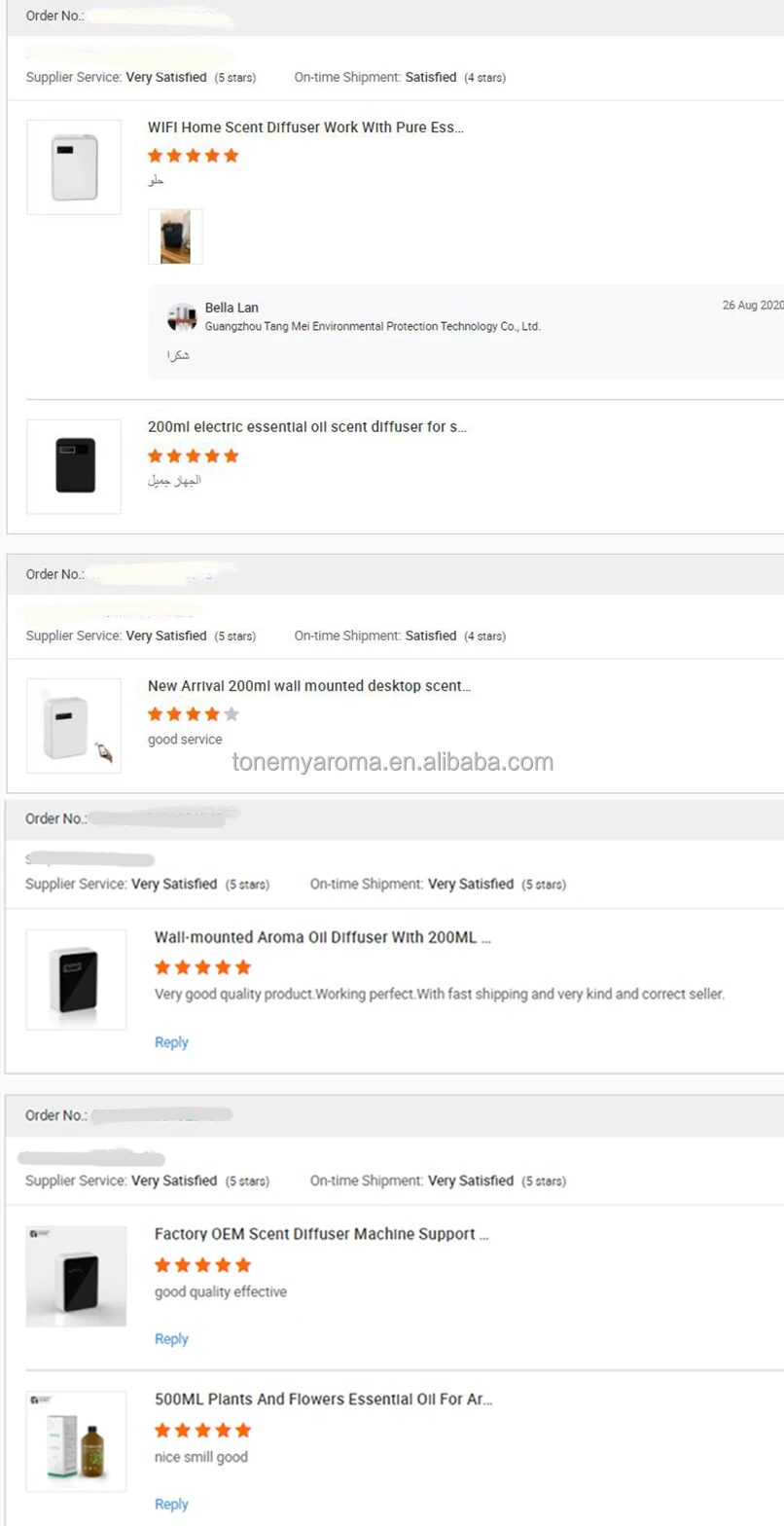The image features a screenshot of a website with a clean, white background divided into three distinct sections. Each section is bordered by light gray bars at the top. The website showcases product information and customer reviews for scent diffusers.

1. **Top Panel:**
   - **Background:** White
   - **Header:** Light gray bar with text "Order Number", the number appears to be obscured by a white mark.
   - **Content:** 
     - "Supplier Service: Very Satisfied (5 stars)" - "Very Satisfied" is in bold.
     - "On Time Shipment: Satisfied (4 stars)"; "Satisfied" is in bold.
     - **Product Details:**
       - "Wi-Fi Home Scent Diffuser with Pure ESS" - partially visible.
       - "Bella Lawn 200 ml Electric Essential Oils Scent Diffuser for S..." - truncated.
     - **Star Rating:** Visible

2. **Middle Panel:**
   - **Background:** White
   - **Header:** Light gray bar with "Order Number", which is blanked out.
   - **Content:**
     - "Supplier Service: Very Satisfied (5 stars)" - "Very Satisfied" is in bold.
     - "On Time Shipment: Satisfied (4 stars)" - "Satisfied" is in bold.
     - "New Arrival: 200 ml Wall Mounted Desktop Scent Diffuser (4 stars)"
     - **Product Details:** 
       - "Good Service"
     - **Star Rating:** Visible

3. **Bottom Panel:**
   - **Background:** White
   - **Header:** Light gray bar with "Order Number", which is blanked out.
   - **Content:**
     - "Supplier Service: Very Satisfied (5 stars)" - "Very Satisfied" is in bold.
     - "On Time Shipment: Very Satisfied (5 stars)" - "Very Satisfied" is in bold.
     - **Product Details:**
       - "Factory OEM Scent Diffuser Machine Support"
       - "500 ml Plants and Flowers Essential Oil for AR..." - truncated
     - **Star Rating:** Visible

Each panel showcases product ratings alongside specific product descriptions and supplier service feedback, emphasizing a strong customer satisfaction rating on key aspects such as supplier service and shipment punctuality.